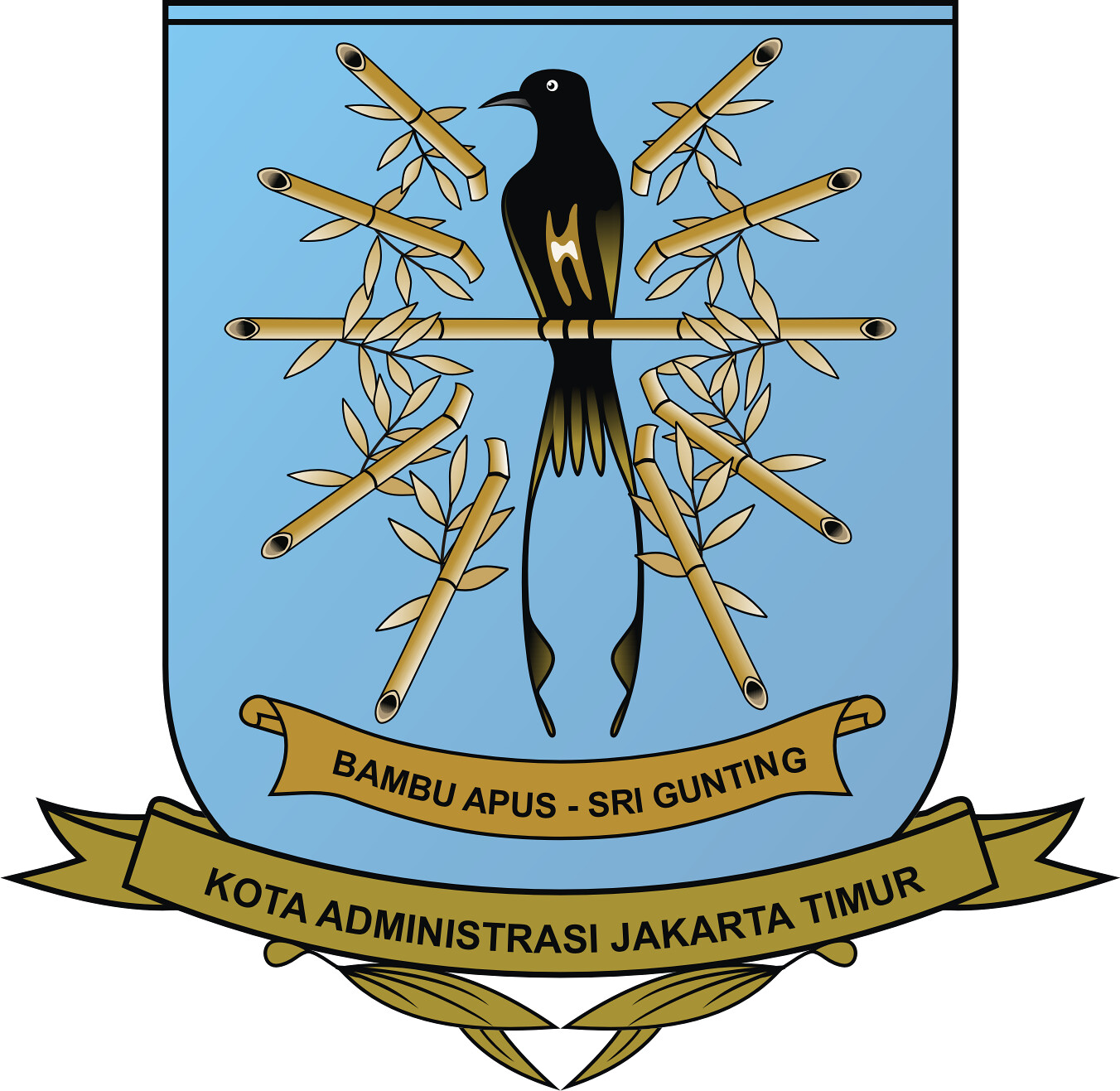This is a detailed, vibrant graphic emblem featuring a sophisticated design. The background is a solid blue shape, flat at the top and sides, curving into a semicircle at the bottom. The emblem is bordered by a black stripe at the very top. At the heart of the design, a striking black bird with brown stripes on its belly and tail is perched on a long, bamboo-like stick. The bird is flanked by bamboo shoots adorned with small brown leaves, which flare both upwards and downwards to the right and left. Below this central imagery, a brown banner with black text reads "Bamboo Apis Sri Gunting," while a similar banner at the very bottom of the blue shape features the text "Kota Administrasi Jakarta Timur," accompanied by brown leaves with black-highlighted veins. The emblem, reminiscent of a soccer team crest or a cultural insignia, combines elements of blue, black, and brown to create a unique and distinguished logo.